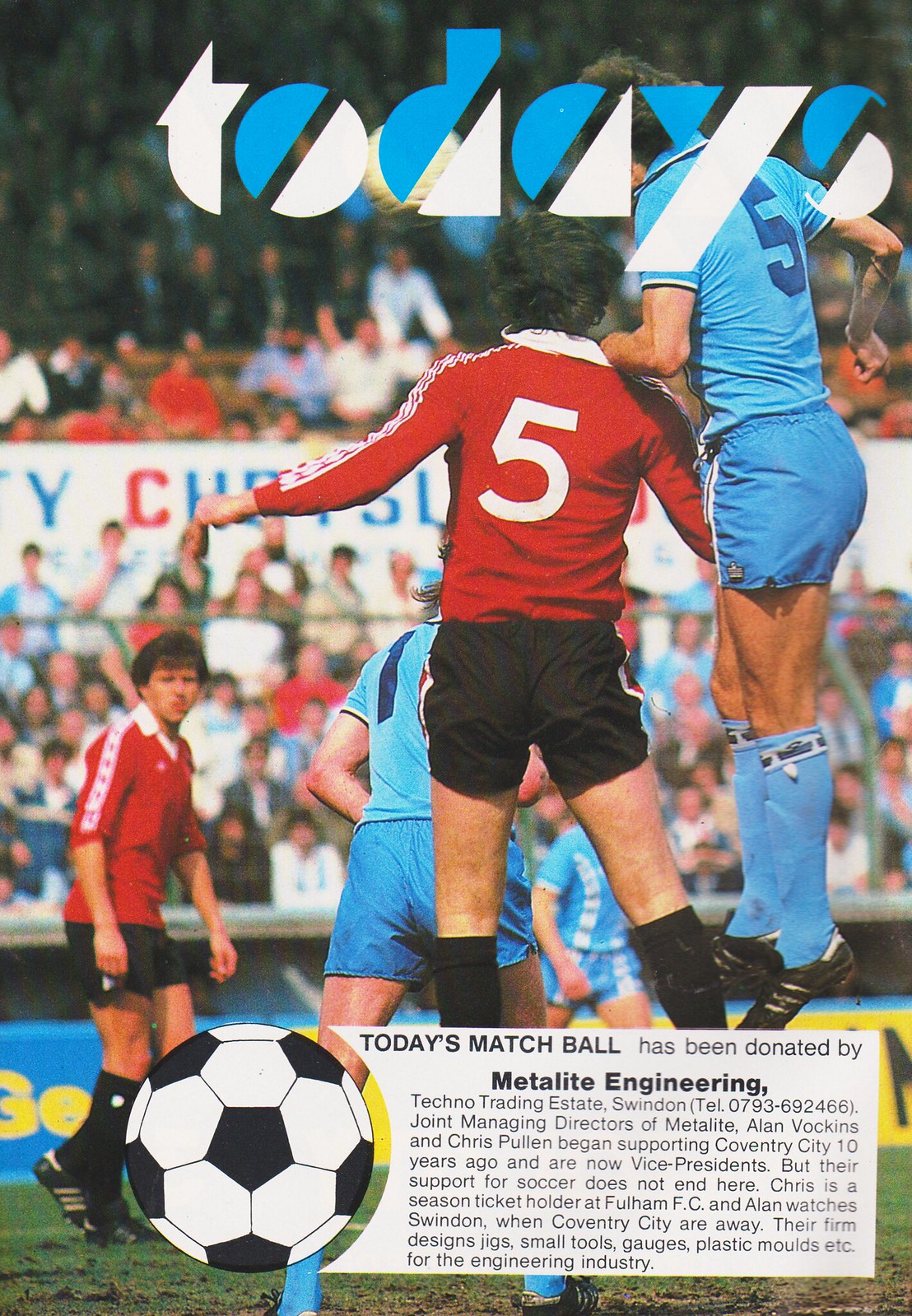The image depicts an older soccer match, likely from the 70s, capturing a dynamic moment on the field. Two players, each from opposing teams dressed predominantly in red and blue, are mid-air, seemingly leaping to head the ball, which is partially obscured behind the headline reading "Today's." The headline is in highly stylized, lowercase font with an upward-pointing oblique line dividing each letter into blue on the left and white on the right. In the center of the image, the focus is on the two players, while other players and a large crowd of spectators are blurred in the background. The setting is a bright, outdoor soccer field. At the bottom of the image, a detailed snippet of text on a white background states, "Today's Match Ball has been donated by Metalite Engineering, Technotrading Estate Swindon, Joint Managing Directors of Metalite, Alan Sockens and Chris Pullen," accompanied by a graphical depiction of a soccer ball. The overall scene is awash in various colors, with green grass, white text, and the vivid red and blue uniforms standing out.